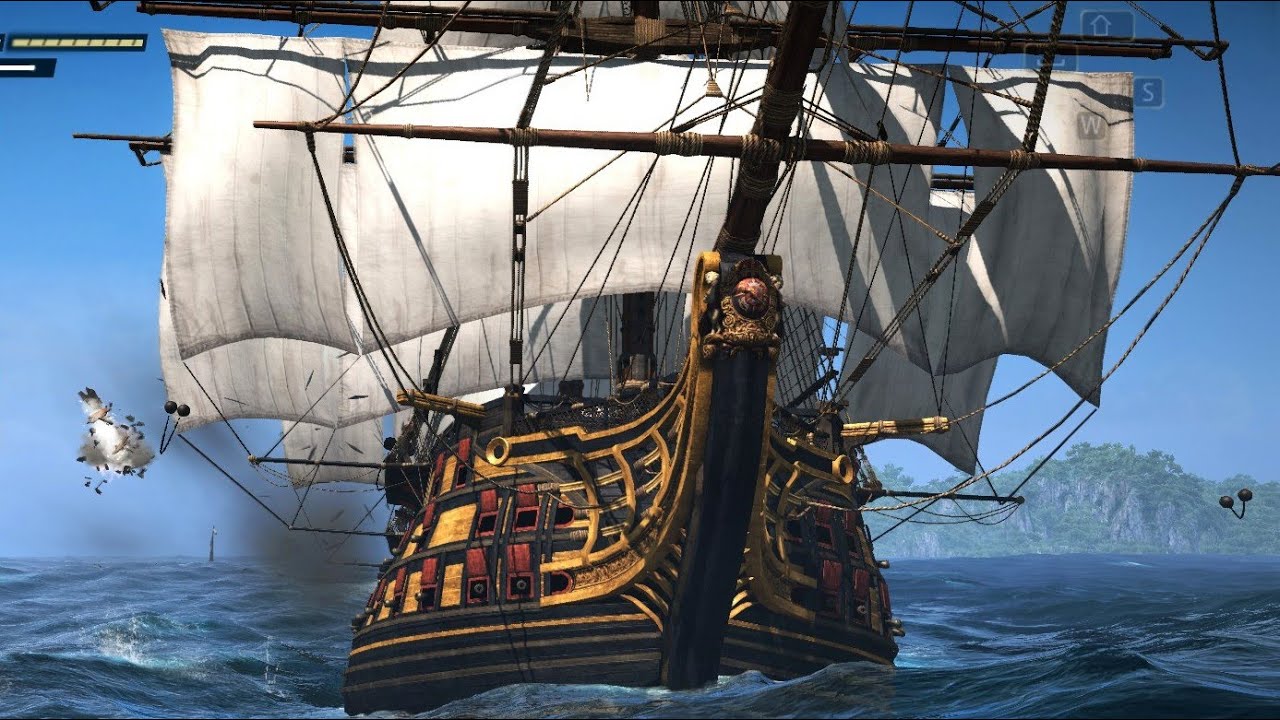This artwork depicts a majestic, intricately designed pirate ship sailing on a vibrant blue sea. The vessel's body is adorned with shades of gold, brown, and dark red, with ornate detailing along its sides. Towering white sails are prominent against the backdrop of a brilliantly blue sky. At the top of the image, a compass displaying 'S' and 'W' can be seen, along with an arrow pointing in a specified direction. The sea itself varies in color, incorporating both dark and light blue hues, enhancing the realistic feel of the water. The setting includes mountains and vegetation in the background, creating the impression of a nearby island. The scene evokes a historical 1800s atmosphere, and while it showcases elaborate details, it retains a somewhat stylized, non-hyper-realistic aesthetic. There are no visible sailors on the ship, suggesting it might be an untouched frame from a video game or a detailed digital painting, capturing the essence of a moment frozen in time.